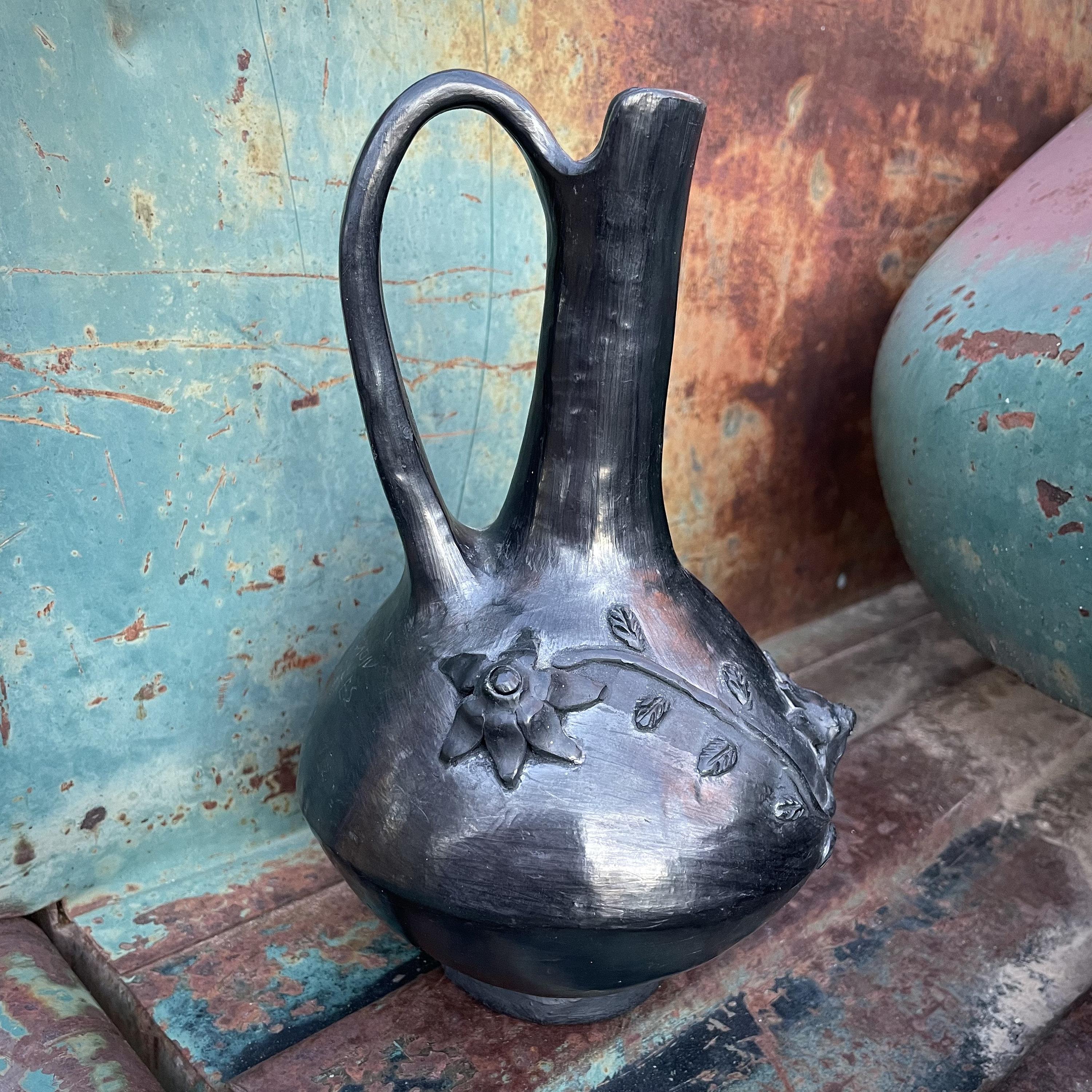The image is a color photograph in a square format, showcasing a striking glazed pitcher as its central subject. This pitcher is meticulously crafted with a rounded bulbous base that gracefully tapers into a slender neck, adorned with an arched handle on the left side. The vessel's surface is a reflective, glossy charcoal black, indicative of glazed ceramic pottery. Intricately engraved on the pitcher is a raised relief image of a flower on a stem, accompanied by leaves on either side, enhancing its visual appeal with floral engravings.

The pitcher is situated on a rustic, weathered shelf that appears to be made of wood, though parts of it have speckled, sprayed paint residues, suggesting it has had various items with ceramic glazes placed on it over time. The shelf and backdrop exhibit a rich patina of multicolored, chipping paint, predominantly showing hues of light eggshell blue and brown rust, hinting at steel that has aged. On the right side of the image, partially visible, is another ceramic object with chipped aqua paint on its lower edge and pink tones near its top, continuing the theme of worn, artistic craftsmanship. The overall composition employs a style of photographic representationalism, capturing the detailed realism of the scene.